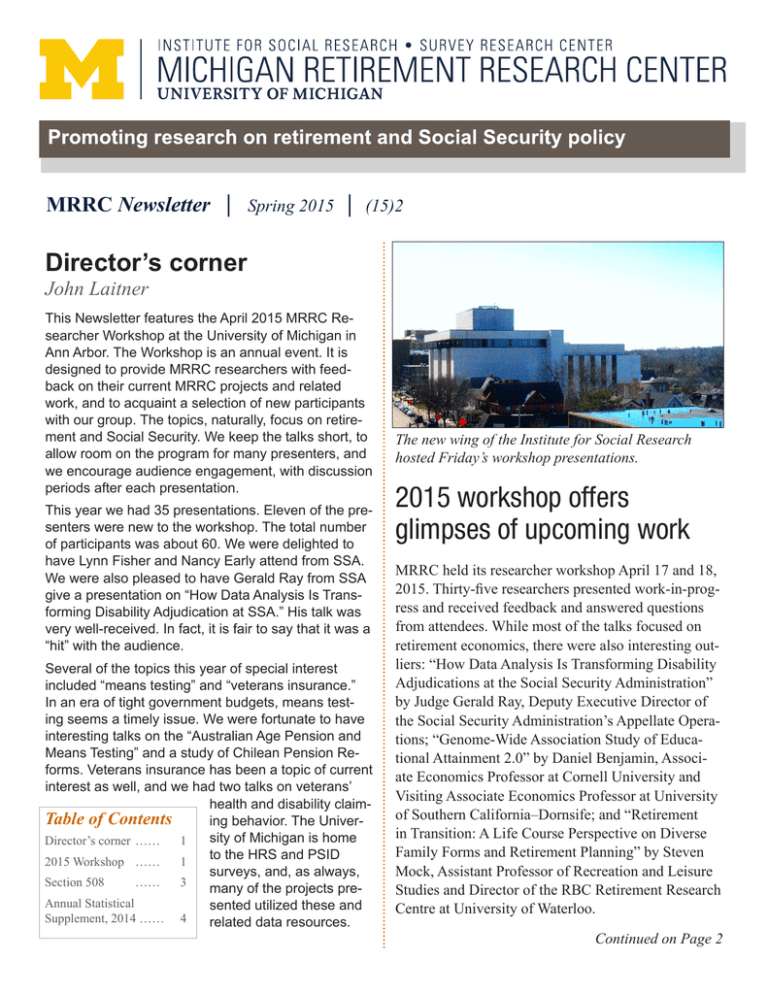The caption for the image should read:

---

At the top left of the image, there is a prominent yellow "M" followed by the text "Institute for Social Research, Survey Research Center, Michigan Retirement Research Center, University of Michigan." Below this heading, in a brownish section, the text reads "Promoting Research on Retirement and Social Security Policy." The center of the image prominently features the title "MRRC Newsletter, Spring 2015," followed by a bold headline "Director's Corner, John Laettner." The content includes multiple paragraphs detailing the newsletter's focus on the April 2015 MRRC Researcher Workshop at the University of Michigan in Ann Arbor. The workshop, an annual event, aims to provide MRRC researchers with feedback on their current projects and related work and to introduce new participants to the group. Topics emphasize retirement and social security, with a format that favors short talks and interactive discussion periods after each presentation. 

At the bottom left of the image, there is a table of contents, and on the right, a picture of a building with the caption "The new wing of the Institute for Social Research hosted Friday's workshop presentations." Below this, additional text announces "2015 workshop offers glimpses of upcoming work."

---